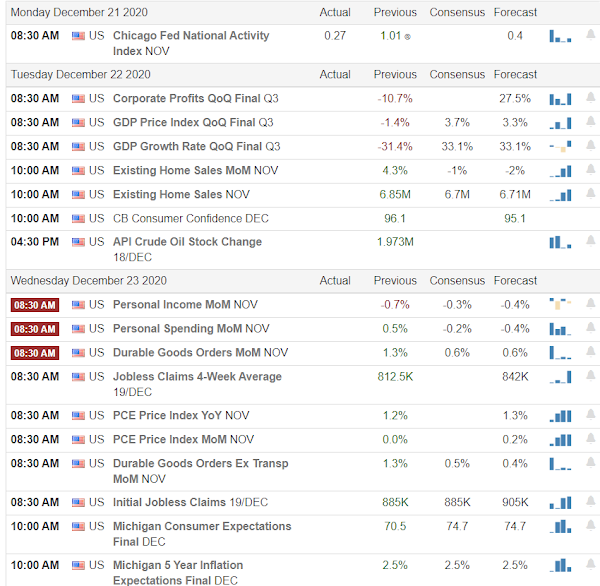The image depicts a comprehensive table detailing various financial markets in the U.S. and their stock statuses over specific dates. At the very top, the table starts with "Monday, December 21, 2020," highlighted with a grey heading and grey bar. Each date features distinct columns for "Actual," "Previous," "Consensus," and "Forecast" values, with the column labels on a white background. 

On December 21, 2020, at 8:30 AM, the table lists the "Chicago Fed National Activity Index, NOV," showing the following figures: an actual value of 0.27, a previous value of 1.01, an empty consensus, and a forecast of 0.4. Accompanying this data is a small graph for visual reference and a notification icon on the extreme right.

Moving to Tuesday, December 22, 2020, the table includes entries like "Corporate Profits, QOQ, Final Q3," "GDP Price Index, QOQ, Final Q3," and "GDP Growth Rate, QOQ, Final Q3."

The last date presented in the table is Wednesday, December 23, 2020, under which several markets are also listed.

Each entry provides a neatly organized snapshot of market performance metrics, essential for investors and analysts tracking changes and projecting future trends.